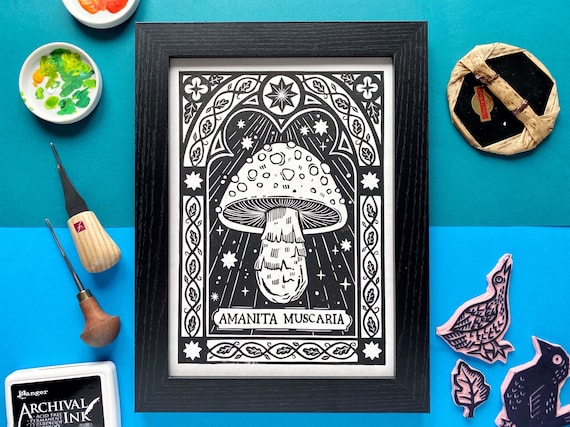The image showcases a black-and-white framed poster of a mushroom at its center, labeled "Amanita muscaria" at the bottom. This detailed drawing features ornate designs, including an archway surrounding the mushroom and white shooting stars in the background. The mushroom itself is adorned with intricate details, such as pebbles or jewels on its cap and a decorative stem. The poster sits on a table covered with two shades of blue tablecloths—robin's egg blue and a darker blue-green hue. Surrounding the poster are various artistic items: white bowls with smeared paint, what appears to be an awl, a leaf and bird cutouts, a shallow wicker basket, and an item labeled "archival ink". The left side of the table features this archival ink item, partially visible with a white outline and black center. Above it are more art tools. Two hand-painted bird cutouts and a painted leaf are also present, with one bird in light pink and black and the other in black. This composition reflects a meticulous and creative setup, blending artistic and natural elements harmoniously.